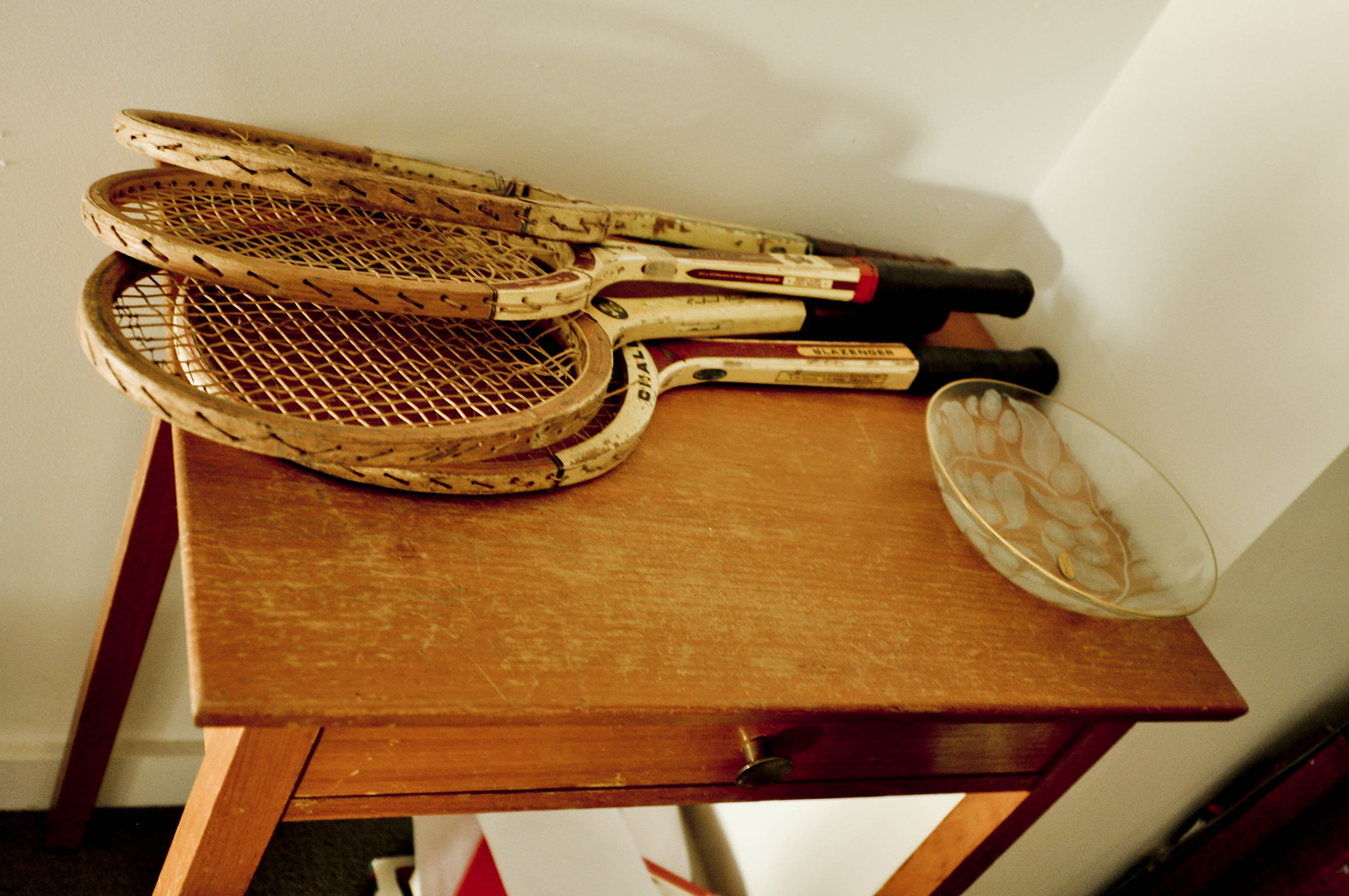In the corner of a white-walled room, a medium-colored, warm wooden table sits, with four sturdy legs and a single long drawer that pulls out. The table appears worn, with scuffs and signs of use. On its right side, a clear glass bowl featuring an ornate floral design and gold trim around the top and bottom rests. Alongside the bowl, four antique wooden tennis rackets with black handles are laid out. The rackets exhibit considerable wear, with chipped paint and frayed webbing, and appear heavily used. Despite their age, the wood at the tops of the rackets is still distinctively lighter in color. The photograph captures a small, intimate corner of the home, hinting at its history through these vintage items.